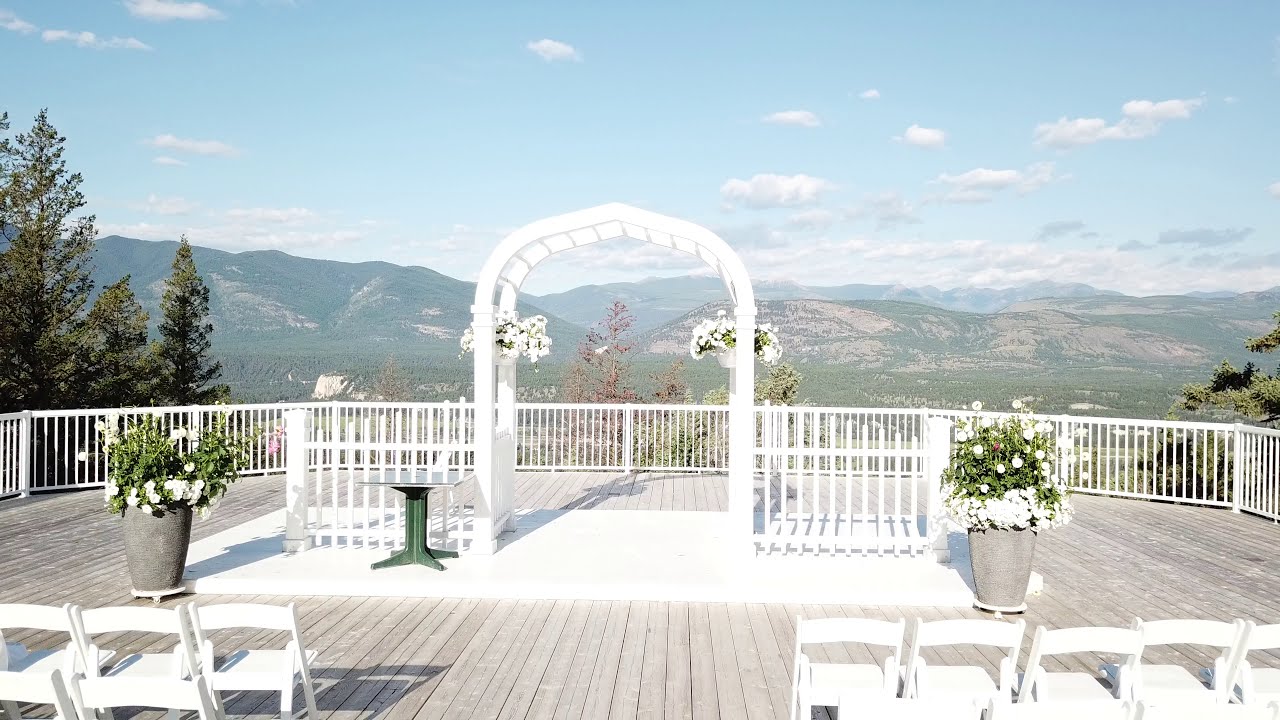This horizontally-aligned rectangular image depicts an outdoor wedding setup on a wooden deck, basking in daytime light. The focal point is a white archway adorned with hanging pots of white flowers, situated on a white rectangular stand. Flanking the arch are two large gray pots brimming with white flowers and lush green leaves. A small table with a green leg and a glass square top stands near the archway. Surrounding the deck, a white fence frames the scene, enhancing the picturesque setting. White folding chairs are arranged in rows on both the left and right, forming an aisle. In the background, the scene overlooks a mountain range, and the sky above is bright blue with scattered puffy white clouds. The left side of the image features some elegant pine trees, while a few branches peek in from the right. The overall image exudes a serene and inviting atmosphere, perfect for a wedding ceremony.